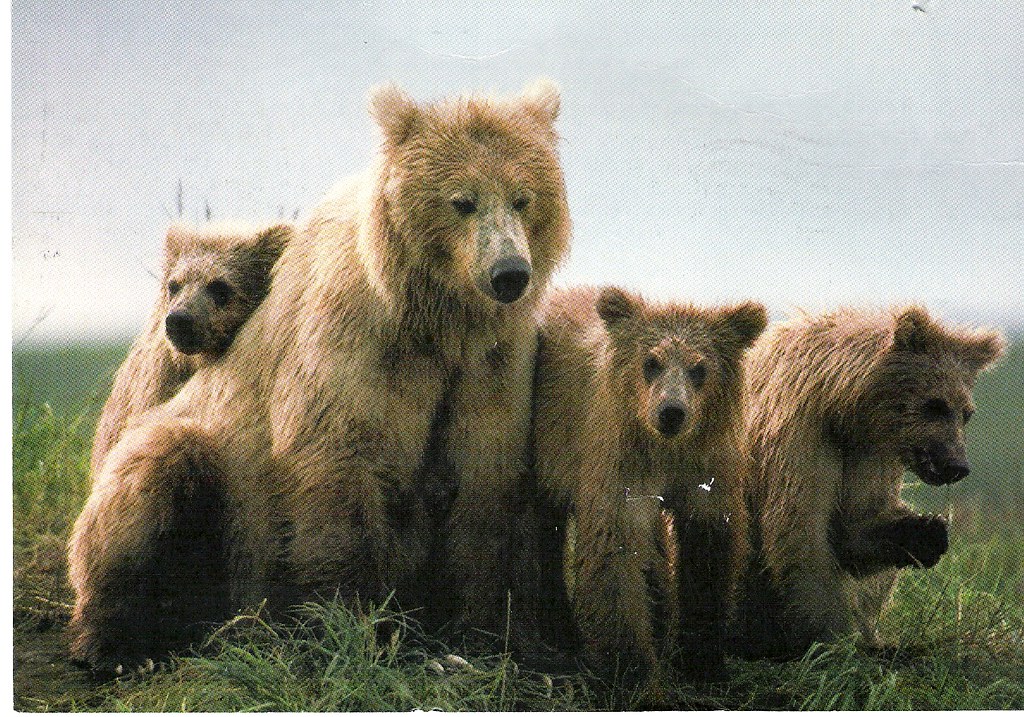In the photograph, which appears to be a well-worn image, possibly from someone's personal collection, a captivating outdoor scene is depicted. Set against a partly sunny sky, transitioning from blue to gray, there is a serene meadow filled with tall, lush green grass. At the heart of this photograph is a family of brown bears — a mother and her three cubs.

The mother bear, positioned on the left side, gazes intently at the camera with a calm demeanor. Nestled close to her, one cub peeks out from behind her back, looking off towards the lower left corner of the image. To the mother bear's right, two cubs can be seen; the first cub is standing on all fours, facing the camera with a curious expression, while the other cub, slightly further to the right, has one paw raised towards its mouth, seemingly eating a piece of grass. The close-knit group visually creates a straight line, all connected with a natural, tender touch, emphasizing the familial bond. Their fur is light tan, harmonizing beautifully with the verdant surroundings, producing an image that exudes both nature's tranquility and the intimate connection between the bears.